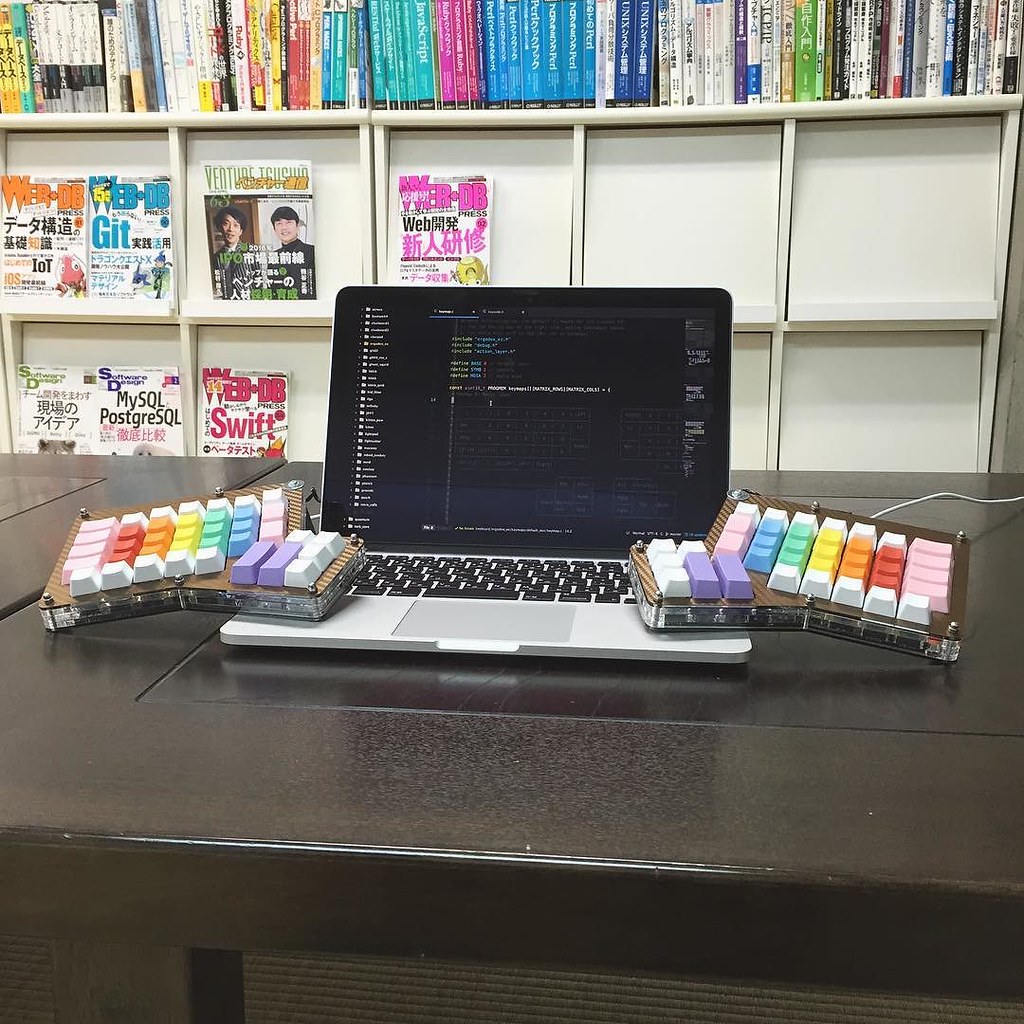This detailed photograph captures an indoor library setting centered around a silver laptop with a black screen displaying indiscernible white text. The laptop, situated on a dark brown table, features additional keyboard panels on either side, adorned with large, multicolored keys in shades of pink, purple, blue, yellow, aqua, orange, and red, suggesting that these might be interchangeable keys for customizing the laptop's keyboard. Behind the table, there is a white bookshelf or magazine rack filled with a variety of items. The top shelf displays an assortment of books with vibrant covers ranging from white to blue, aqua, pink, yellow, and red. On the left-hand side of the bookshelf, several magazines, presumably in an Asian language and featuring Asian men, are prominently displayed. The bottom part of the shelf is noted for its organized rows of items, potentially DVDs, with their titles clearly visible.